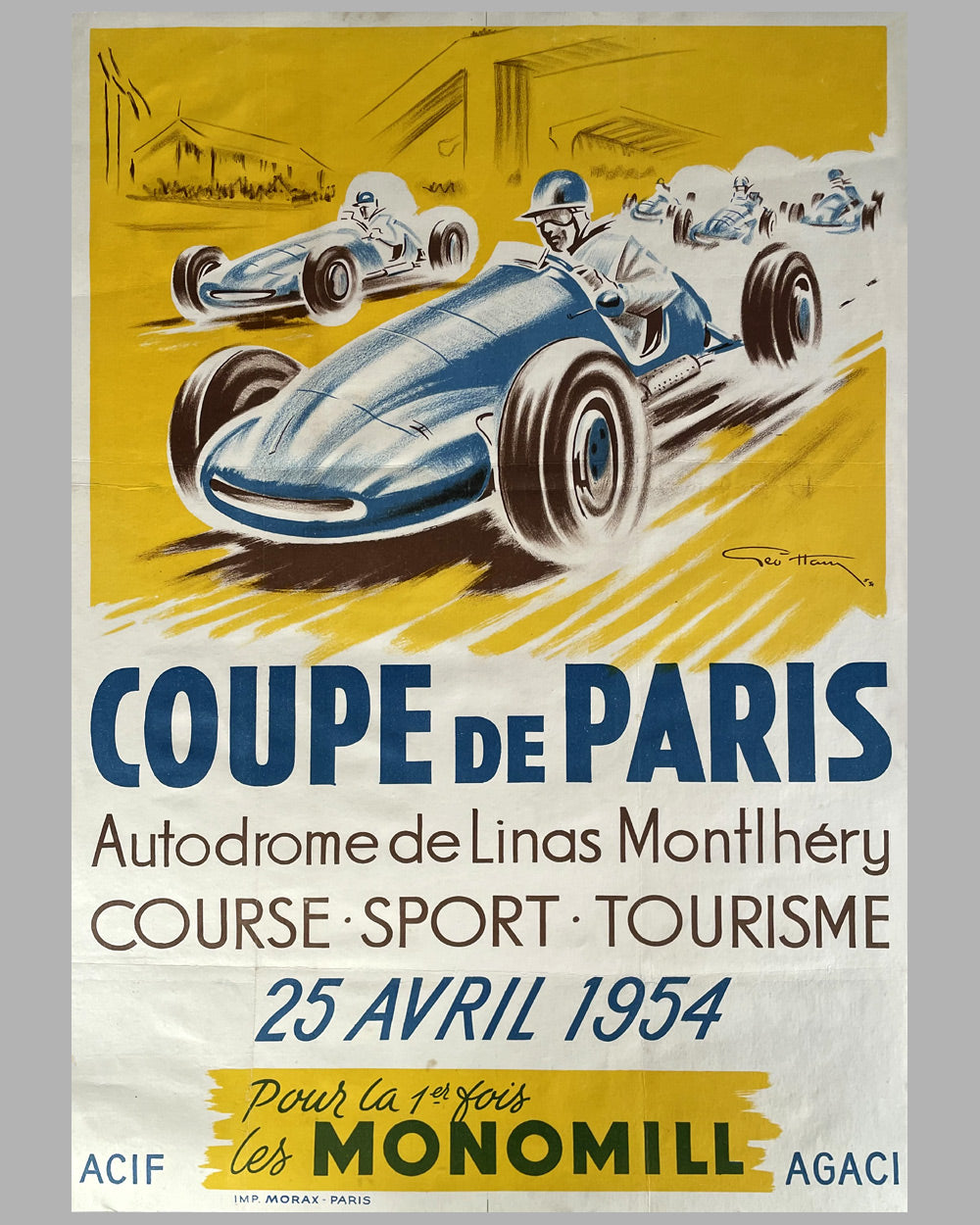This detailed vintage poster, designed for a 1954 car racing event, features a striking illustration in blue and yellow. It portrays a thrilling race with vintage blue cars, each with four black tires and open cockpits, where helmeted drivers are racing towards the left side of the image. The cars are depicted low to the ground on a yellow track, with a charcoal sketch of an overpass and a building in the background, adding depth to the scene. Surrounding the central image is a white border with further text details. The bold blue text at the bottom reads, "Coupe de Paris," followed by "Autodrome de Linas Montlhéry" in black text. Beneath it, in uppercase, are the words "COURSE SPORT TOURISME," and the date "25 Avril 1954" is prominently featured in bold dark blue. The entire poster is framed by a thin grey border, set against a grey background, giving it a classic and timeless aesthetic.